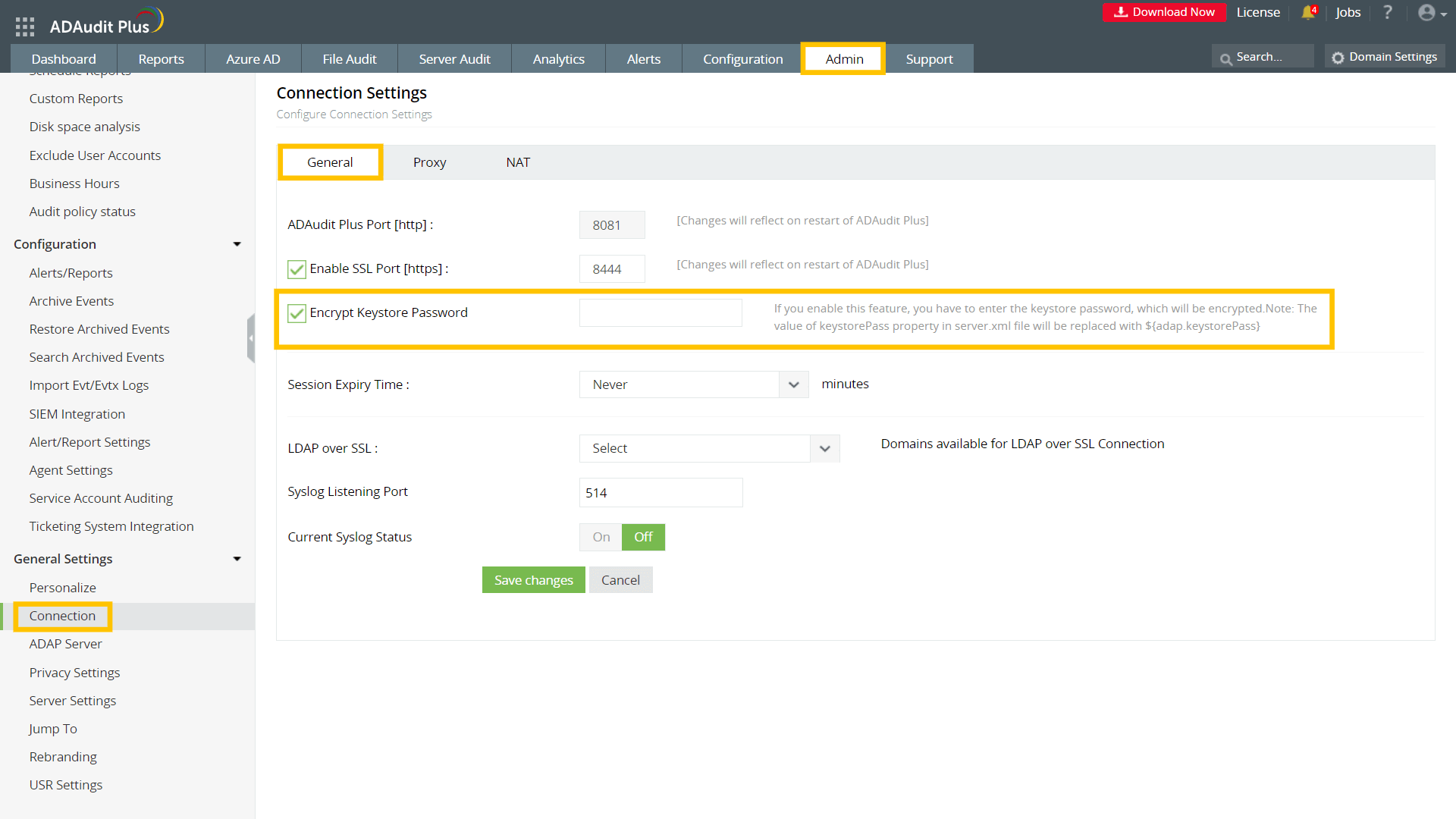Here’s a cleaned-up and detailed caption for the image:

---
Screenshot of the "Add Audit Plus" program interface displaying various navigation options. The left side features a vertical gray bar with multiple configuration options, while the main area shows tabs and submenus. The primary tab labeled "General" is highlighted with a yellow circle, indicating the active section. Within this section, the submenu item, which appears to be "Encrypt Key" or "Keystroke Password," is also circled in yellow. Below this, four additional options are visible but too small to be legible. At the bottom of the screen is a prominent green "Save Changes" button. The comprehensive main menu includes entries for Dashboard, Reports, Access ID, The Audit, Server Audits, Analysis, Alerts, Configuration, Admin, and Support.

---